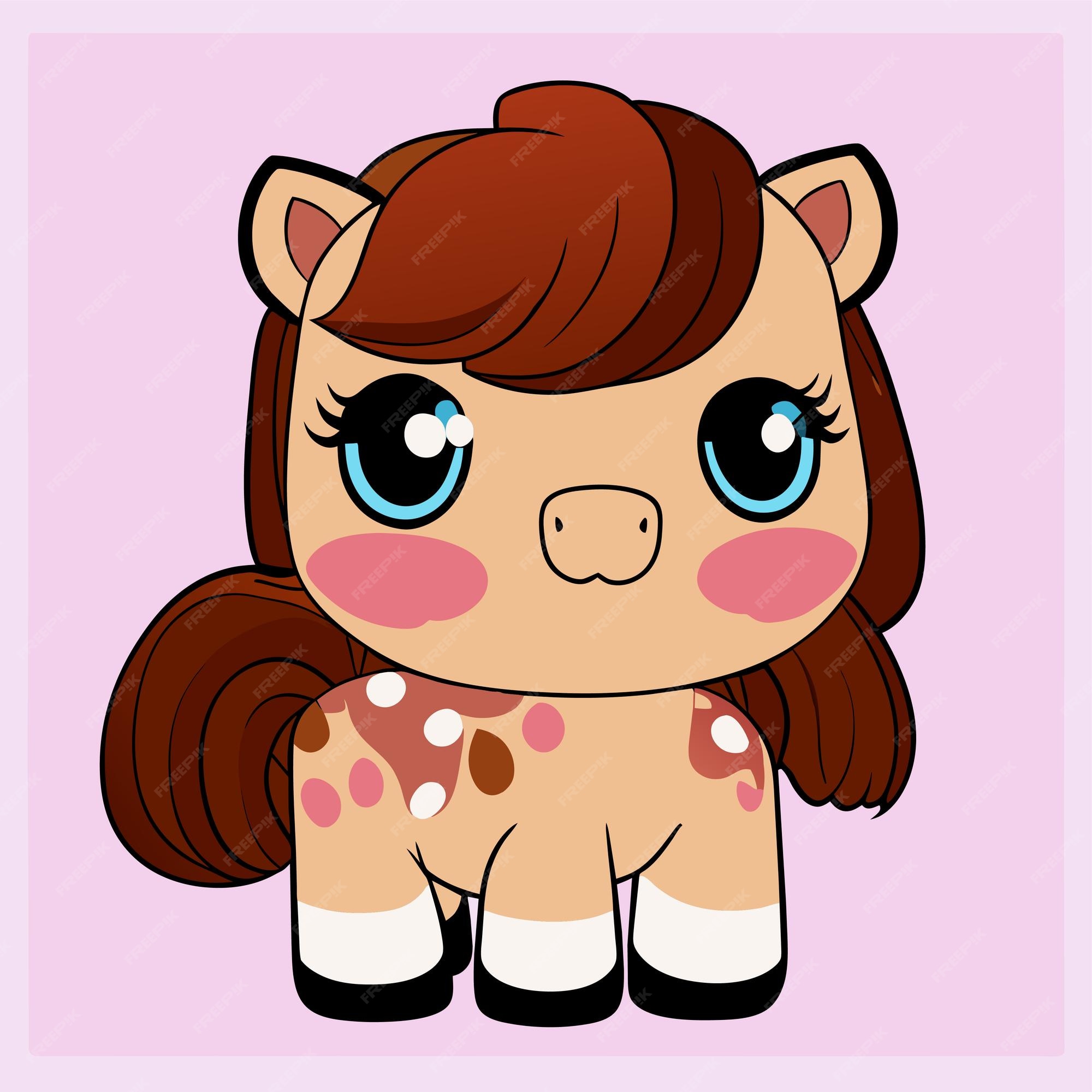This image features a chibi-style cartoon pony reminiscent of My Little Pony, set against a pink background. The pony has a tan-colored body adorned with pink, brown, and white spots. Its hooves are black with a white stripe directly above them on all four legs. The pony’s face is peach-colored with rosy cheeks and a pronounced snout featuring two black nostrils. Its large, expressive eyes are black with a blue ring around the bottom and white dots at the center, with three eyelashes on the left eye and four on the right. The auburn mane with dark brown strands sweeps across the forehead and cascades down the back, while its ears, which have a black outline, are flesh-colored on the inside with a pink section. The entire image is overlaid with a faint gray watermark that says "freepik" repeated diagonally. The overall appearance is cute and meant for a child-friendly design, likely for a cartoon or comic aimed at young girls.